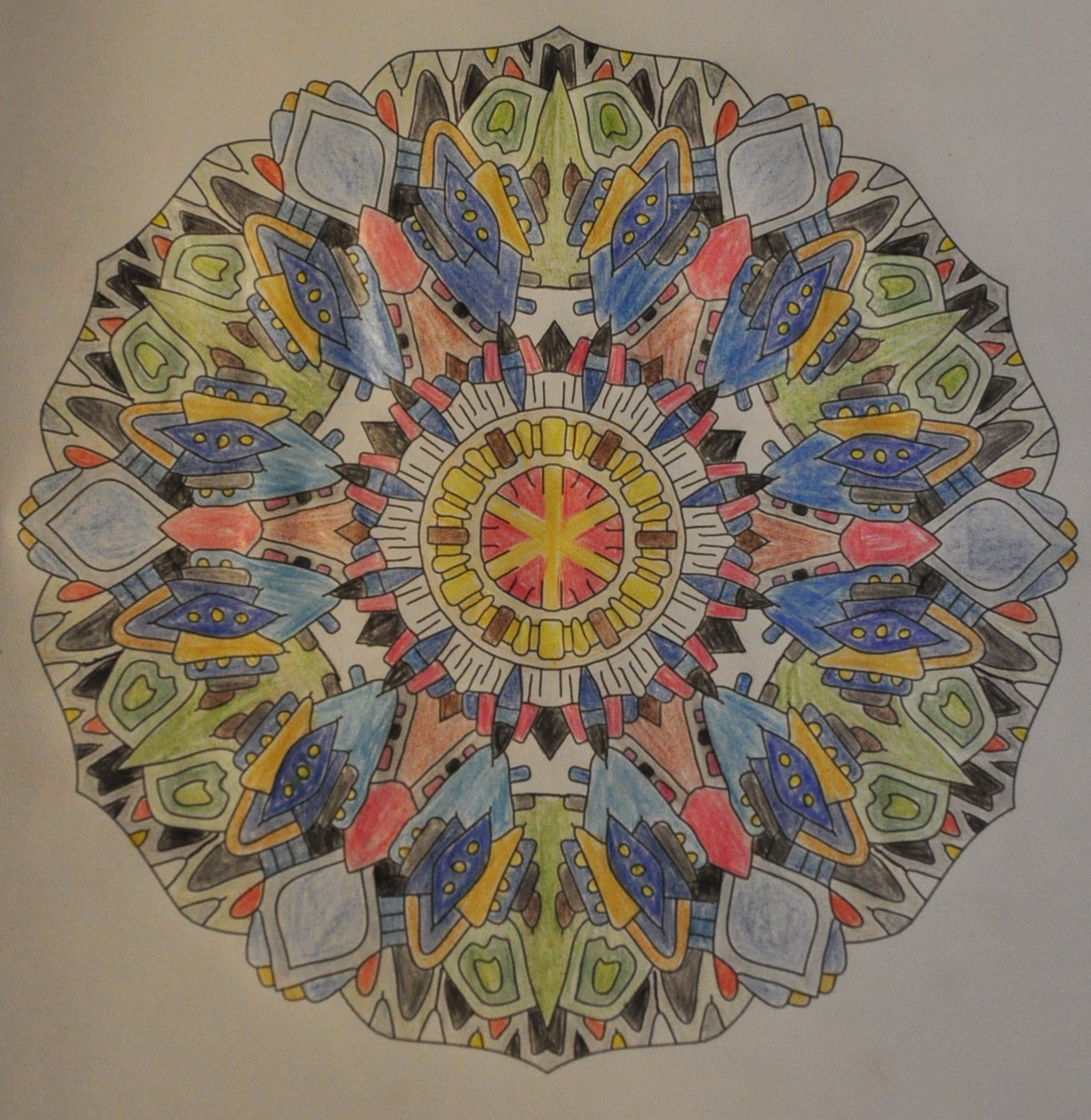This square image showcases a vibrant, hand-drawn mosaic set against a white background. At its center lies a smaller circle adorned with intricate decorations, predominantly colored in red with yellow crosshair-like details. Surrounding this central circle, the mosaic features an array of tiny drawings and shapes, each meticulously filled with a multitude of colors, likely applied using crayons or colored pencils. The outer section of the mosaic seems to be bordered by stone-like elements, enhancing its intricate design. While not every section is colored in, the majority of the mosaic bursts with diverse, vivid hues, creating a rich and intricate visual tapestry.